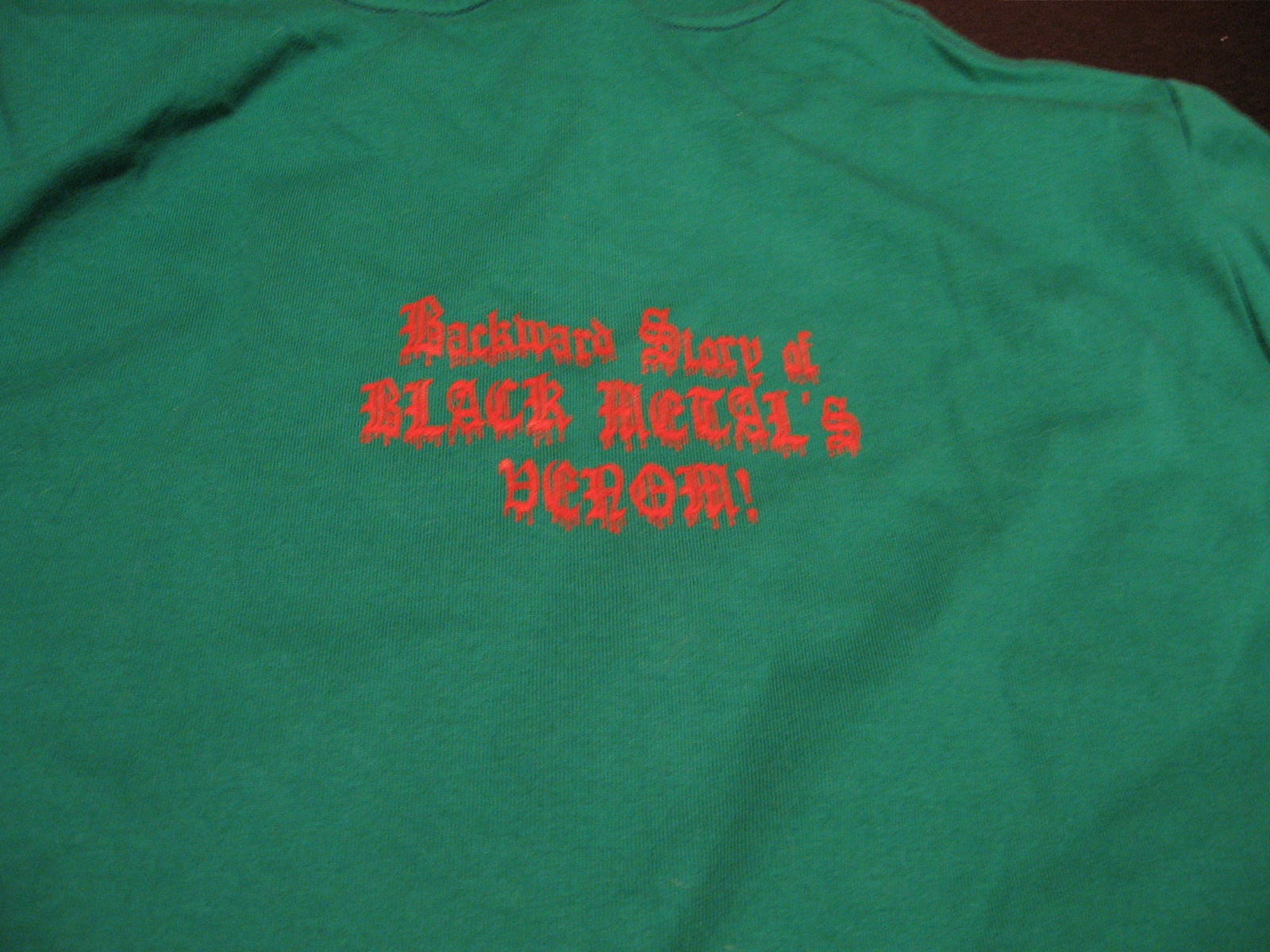The image is a wide rectangular picture, primarily depicting a piece of green fabric that might be the back of a T-shirt. In the upper right-hand corner, there's a small area of brown, hinting at a surface beneath the fabric. Dominating the center of the green fabric is red text in Gothic lettering, which can be challenging to read. 

The top line reads "Backwards Story Of," with the 'B' and 'S' capitalized. The second line is in all uppercase letters and reads "BLACK METAL'S." The bottom line appears to start with "DEA," followed by two ornamented letters. The second-to-last letter is a circle with a line and a cross in the middle, resembling a stylized 'T'. The final letter looks like an 'M' with a horizontal line through it, and the line concludes with an exclamation point.